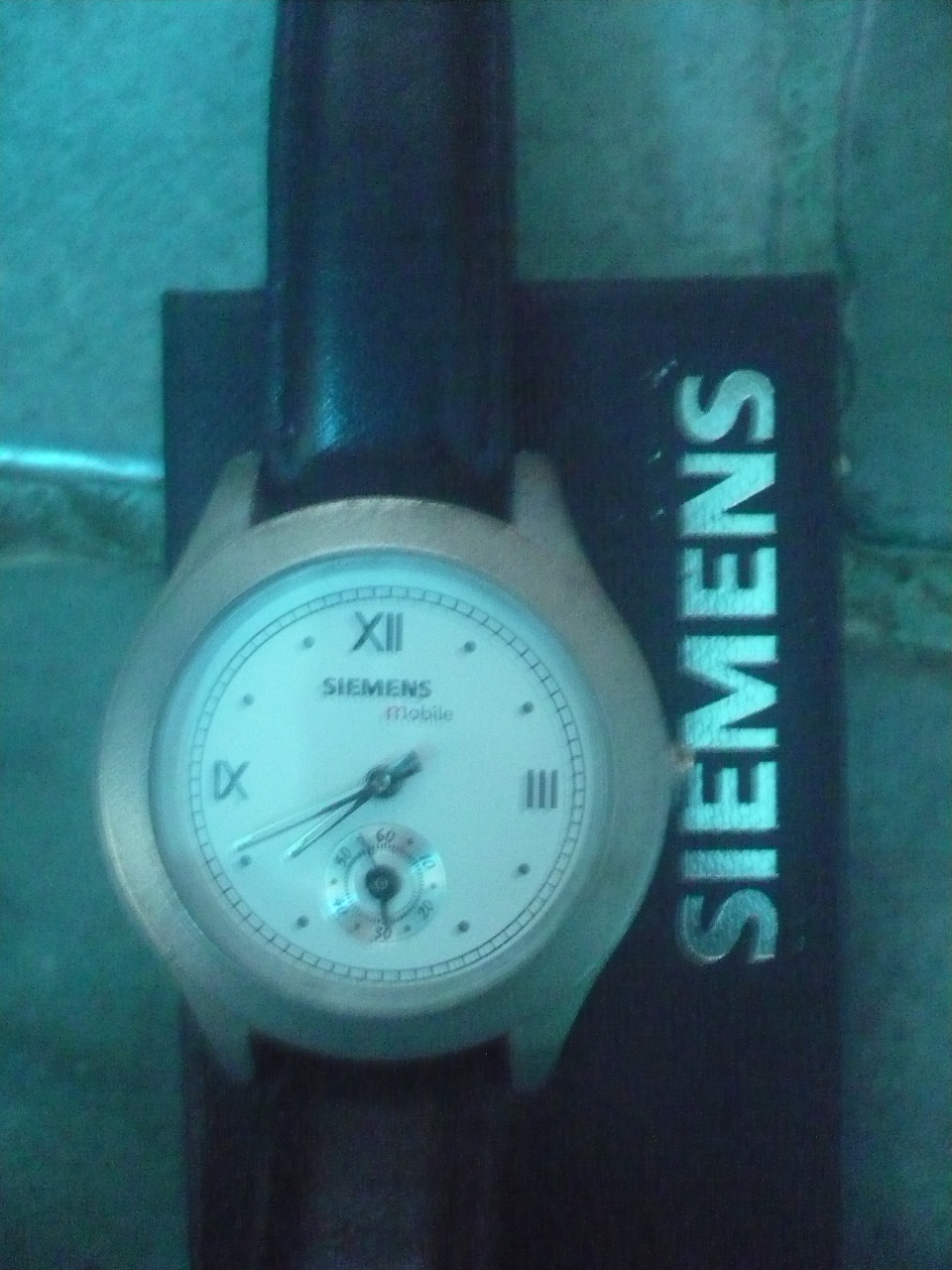This evocative image showcases a sophisticated wristwatch against a moody, bluish-dark backdrop. The watch features a black leather band that exudes elegance and durability. The bezel of the watch is a light, likely metallic, color, providing a striking contrast against the dark-themed setting. The watch face is pristine white, adorned with a minimalist design. Encircling the face, there is a double-lined circular border that adds a touch of refinement. Positioned vertically and dividing the watch face exquisitely are hour markers at 12, 3, and 9, indicated by Roman numerals XII, III, and IX, respectively. Notably, at the 6 o'clock position, there is a smaller sub-dial with its own set of markers ranging from 10 to 60, likely for seconds or an alternate timekeeping function, with a delicate hand pointing to these subdivisions. The attention to detail in the design and the ambiance of the image truly highlight the craftsmanship and style of this timepiece.